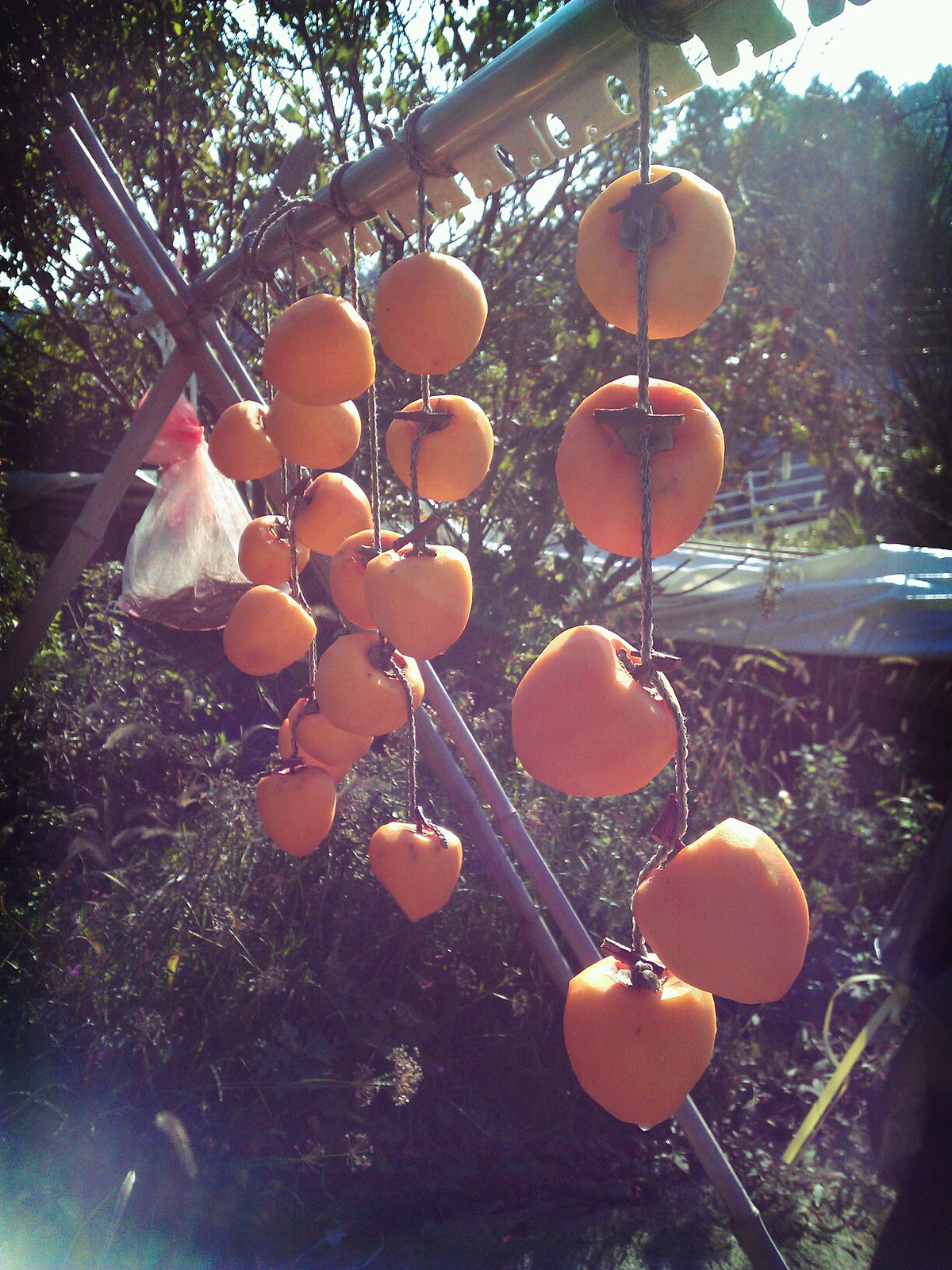This photograph captures a vibrant outdoor scene, likely taken in the afternoon as evidenced by the sunlight filtering through the trees and casting a warm glow. The focal point is a makeshift drying rack constructed from bamboo poles, designed with a metal frame forming an X-shape reminiscent of a tipi structure, from which strands of fruit are suspended. The fruits, possibly peeled mangoes, apples, or even apricots, are tied together on strings, each strand holding about five to six pieces. The fruits exhibit a peach or orange hue, though there is some debate on their exact type, as they could be peppers or even artificial. To the left, a plastic bag filled with an unidentified substance hangs precariously, likely from a tree branch obscured by the foliage. Surrounding the scene are various shrubs, bushes, and a patch of green grass, with a white fence and a road visible in the distance. The sunlight dapples through the canopy, emphasizing the lush greenery and creating a serene garden atmosphere.